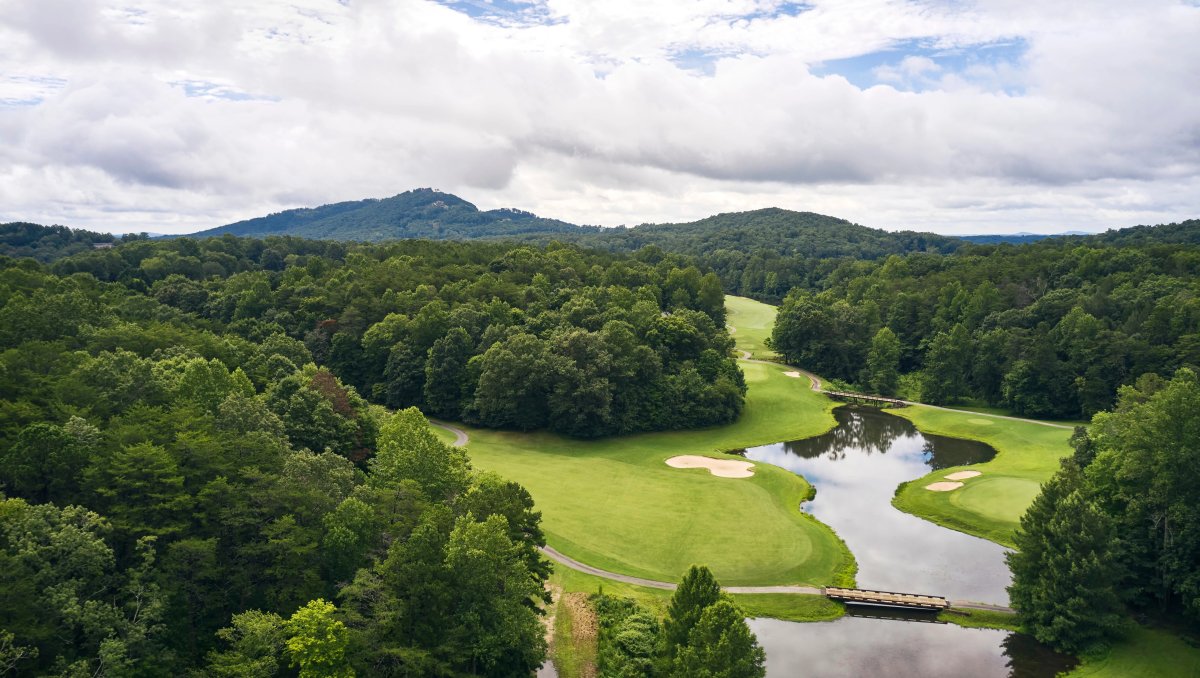This aerial photograph captures a serene, well-manicured golf course nestled within a dense, expansive forest. The scene is dominated by lush green grass and dotted with several sand traps, including one on the left side of a calm, winding river and two more on its right. A small walking bridge spans the river, connecting various paths that meander through the landscape, evidently designed for both hikers and golfers. Another bridge can be seen further in the background. The golf course is framed by a large grove of trees on both sides, creating a picturesque contrast against the manicured grounds. In the distance, wooded hills rise up, thick with trees, adding depth to the image. Above, the sky is filled with a mixture of fluffy white clouds and patches of blue, hinting at a tranquil, possibly overcast day, with the potential for rain hidden within the subtle gray shades of some clouds. The overall impression is one of peace and natural beauty, with no visible human activity, making the scene calm and inviting.